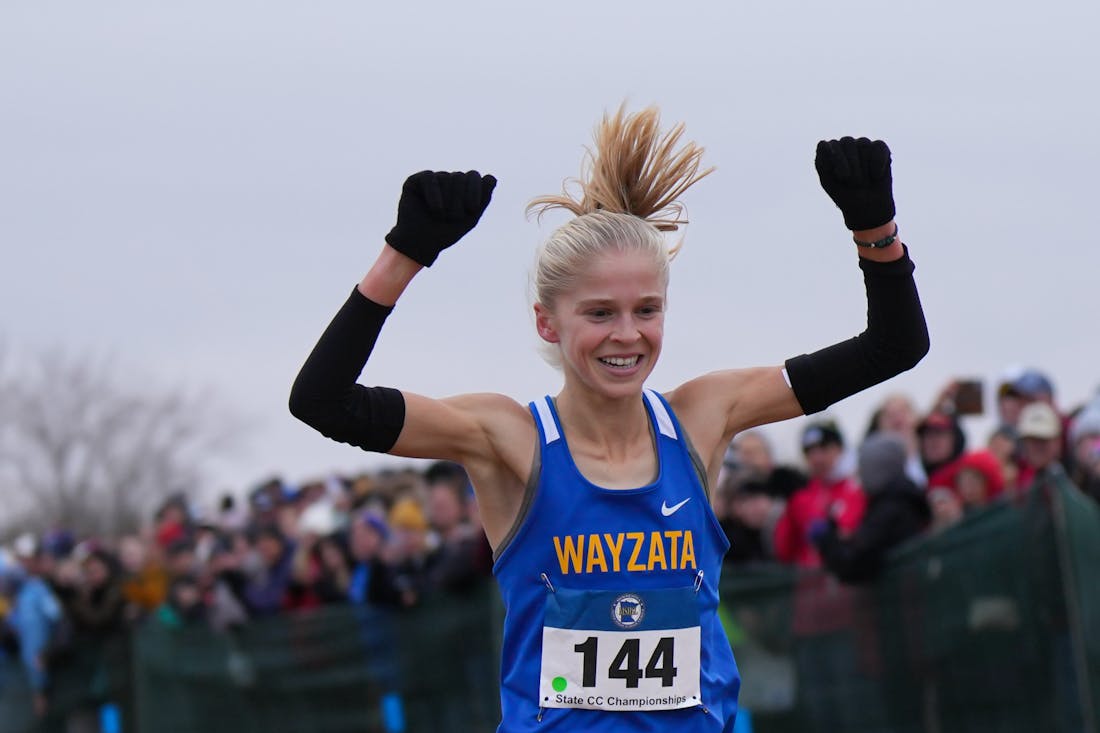This is a detailed photograph of a young, slim, and muscular female athlete, likely a long-distance runner, who appears to have just completed a race. She radiates happiness and enthusiasm, her broad smile reflecting her joy at possibly finishing in a top position. Her arms are raised in a triumphant gesture, hinting she may have crossed the finish line. She has blonde hair tied in a ponytail that is flicked up in the air, emphasizing her recent movement.

She is attired in a blue tank top jersey with a prominent white Nike logo on the left side. In bold yellow capital letters, the word "Wayzata" is displayed across the front, and below it, a white bib with the number 144 and the words "State CC Championships" is pinned on, where "CC" likely stands for cross country. To keep warm on this cold day, as suggested by the warmly dressed crowd and the gray, overcast sky, she wears black gloves and black arm protectors that cover from her wrists to the middle of her biceps. On her left wrist, she sports a black watch.

In the background, the cheering crowd is captured out of focus, standing behind a green shade cloth barrier. Their presence and the barren trees hint at the chilly weather, further supported by the athlete's warm attire. The entire scene is set outdoors, creating a vivid picture of a championship moment.